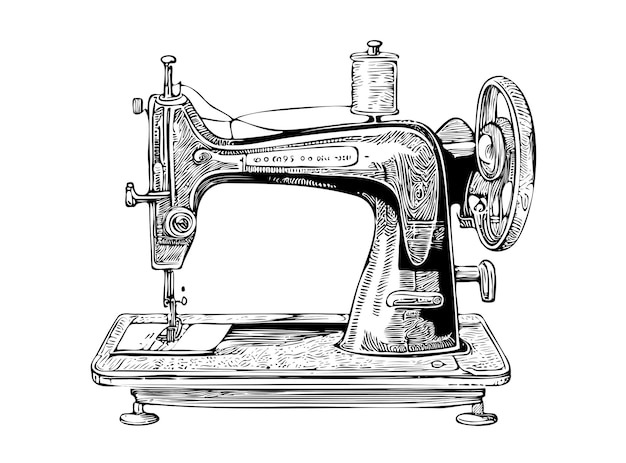This detailed black and white illustration depicts a classic, old-style sewing machine on a pure white background. The sewing machine features a rectangular base with slightly curved corners and feet that resemble suction cups. Prominently placed on top is the spool of thread, positioned towards the right side, with the thread feeding into the machine and down into the bobbin. The right side of the sewing machine displays a large wheel, accompanied by a handle and multiple levers. Despite some small, nearly unreadable imprints which may indicate the name or serial number of the machine, the image exudes a simplicity often seen in patent application drawings, emphasizing the machine’s timeless, utilitarian design.